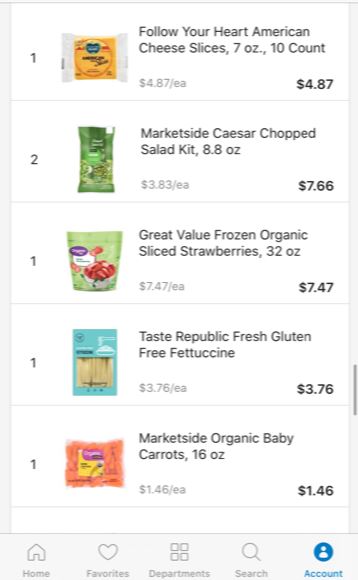Here is a cleaned-up and detailed caption for the described image:

---

This image is a screenshot of an online store. The background is white, with text displayed in black, although the image is slightly blurry. The store features five different products:

1. **Follow Your Heart American Cheese Slices**:
   - **Quantity**: 7 ounces, 10 count
   - **Price**: $4.87 each
   - **Product Description**: The cheese slices are yellow and displayed on the left side of the screen.

2. **Marketside Caesar Chopped Salad Kit**:
   - **Quantity**: 8.8 ounces
   - **Price**: $3.83 each
   - **Total Price**: $7.66 (since there are two of these in the cart)
   - **Product Description**: The salad kit is depicted on the left side, showing that two units of this product are in the shopping cart.

3. **Great Value Frozen Organic Sliced Strawberries**:
   - **Quantity**: 32 ounces
   - **Price**: $7.47 each
   - **Product Description**: The package is green with images of red strawberries, and one unit is shown on the left.

4. **Taste Republic Fresh Gluten-Free Fettuccine**:
   - **Quantity**: Not specified
   - **Price**: $3.76 each
   - **Product Description**: The packaging is light blue and brown, shown on the left side.

5. **Marketside Organic Baby Carrots**:
   - **Quantity**: 16 ounces
   - **Price**: $1.46 each
   - **Product Description**: The carrots are orange and depicted on the left. 

The bottom of the screen shows the navigation bar featuring the icons:
- **Home**
- **Favorite**
- **Department**
- **Search**
- **Account**

The "Account" icon is highlighted in blue on the bottom right.